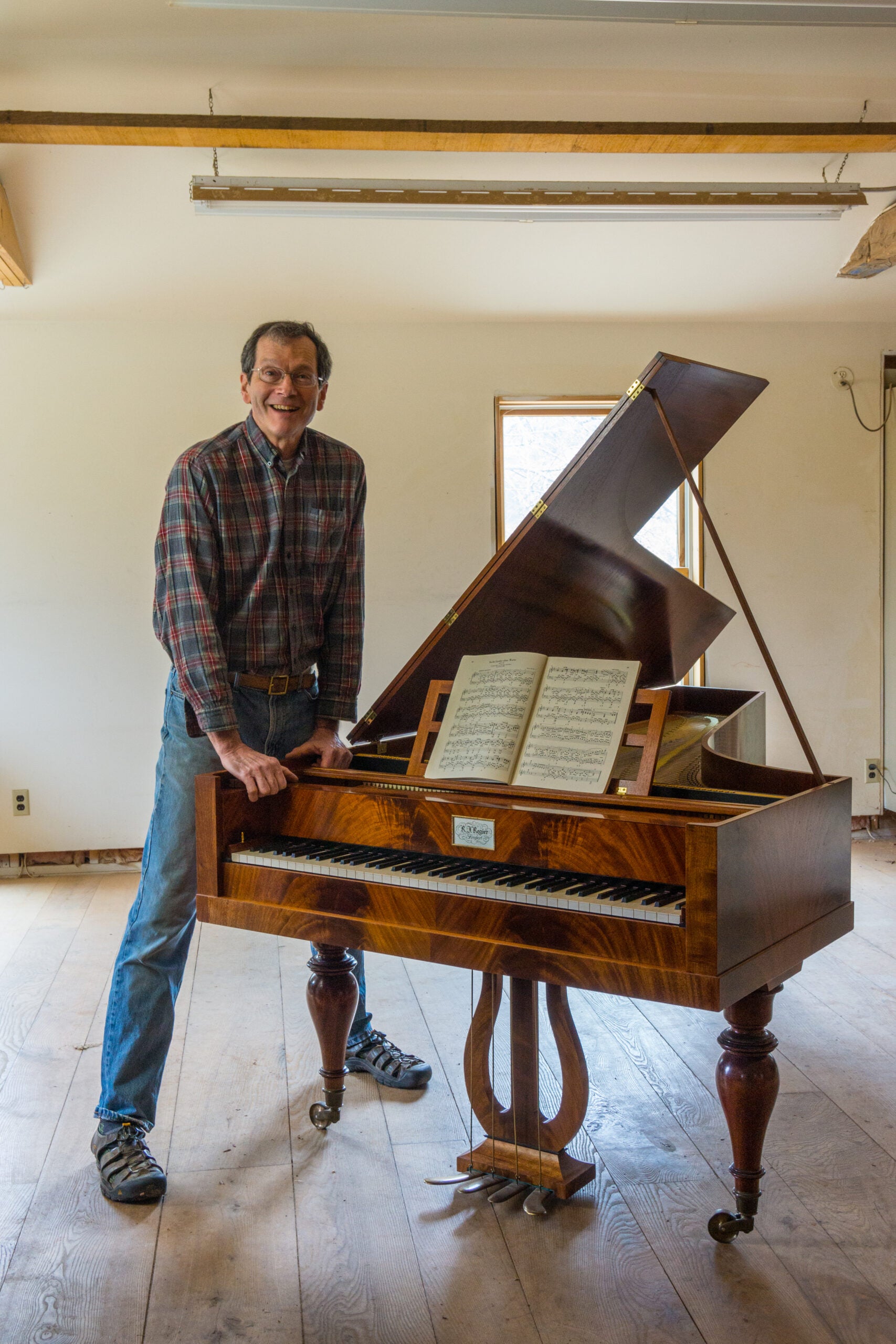A detailed real-life photograph depicts an older man standing next to a large, elegantly crafted piano. The piano, constructed with a dark-stained wooden frame, stands prominently with its two front legs visible and an ornate column at the center, presumably where the pedals are attached. The view from the front reveals the black and white keys, along with a holder for sheet music. The piano lid is propped open by a stick, showcasing its grandeur.

The man, dressed in a plaid shirt and jeans, is positioned to the left of the piano. He has dark gray hair and wears glasses. His stance is casual, with legs slightly spread and gripping the piano as he leans against it. Behind him, the room's white walls contrast with several exposed wooden beams, and the floor consists of old, worn-out wood, giving an impression of an ongoing renovation project in the house.